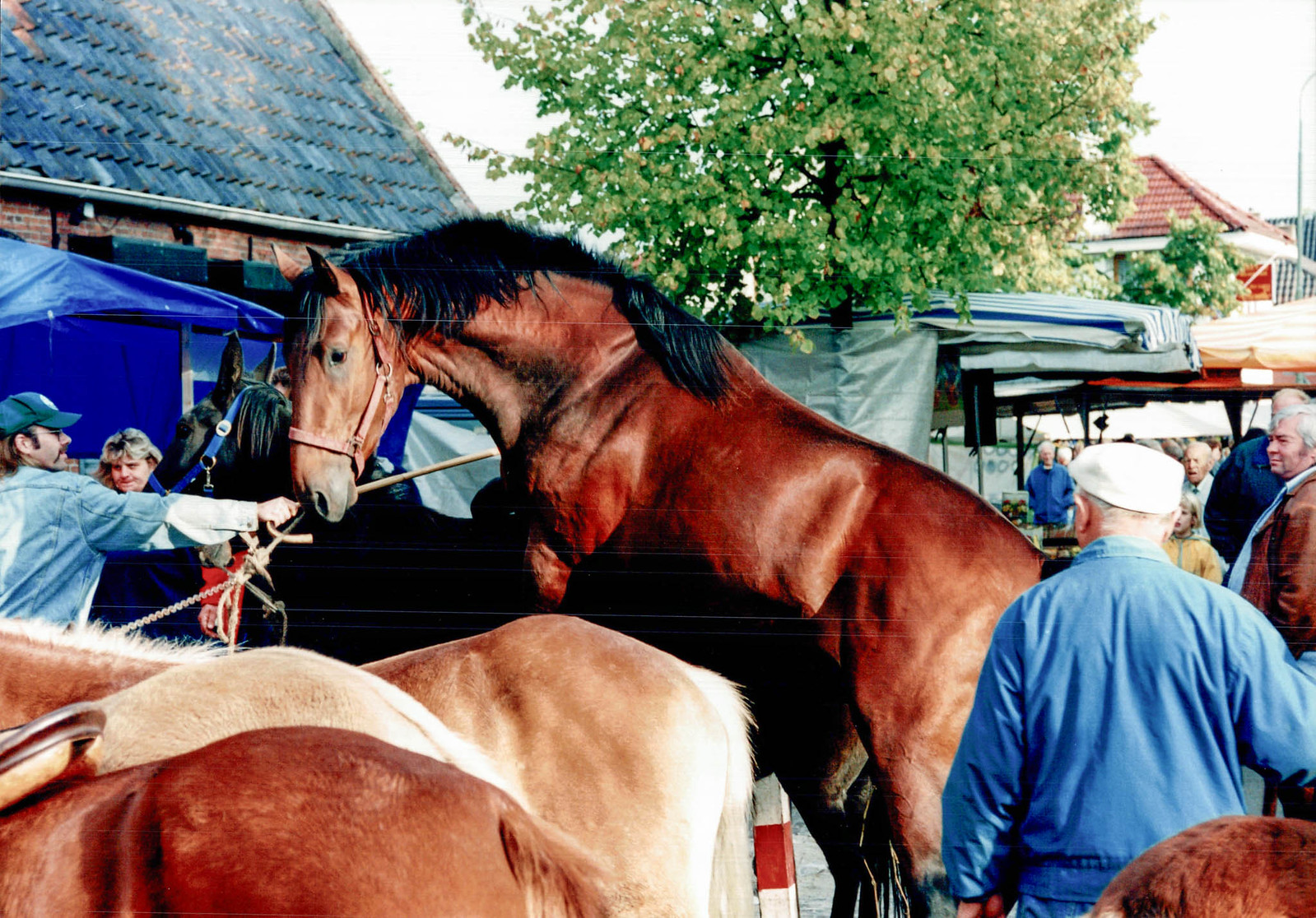This outdoor photograph captures a vivid scene of a horse mating process. Dominating the center of the image is a large brown horse with a black mane, rearing up on its hind legs while its front hooves rest on the back of a black horse, signifying the stud mating with the mare. Both horses are equipped with harnesses, with the black horse's harness being notably blue. In the foreground, the rear ends of three additional horses are visible, with another partial horse visible on the lower right. There is a man in the immediate foreground, his back turned to the camera, wearing a blue jacket and a white Jeff cap. To the left, another man in a denim jacket and blue hat is holding a rope connected to the harness of the rearing horse. This bustling scene is surrounded by several other people who appear to be observing the event, possibly at a county fair or similar outdoor exhibit. A large tree stands centrally behind the horses, and in the background, a building with a slate roof and a blue tarp can be seen. The bright daytime sky illuminates the scene, ensuring all details are clearly visible.